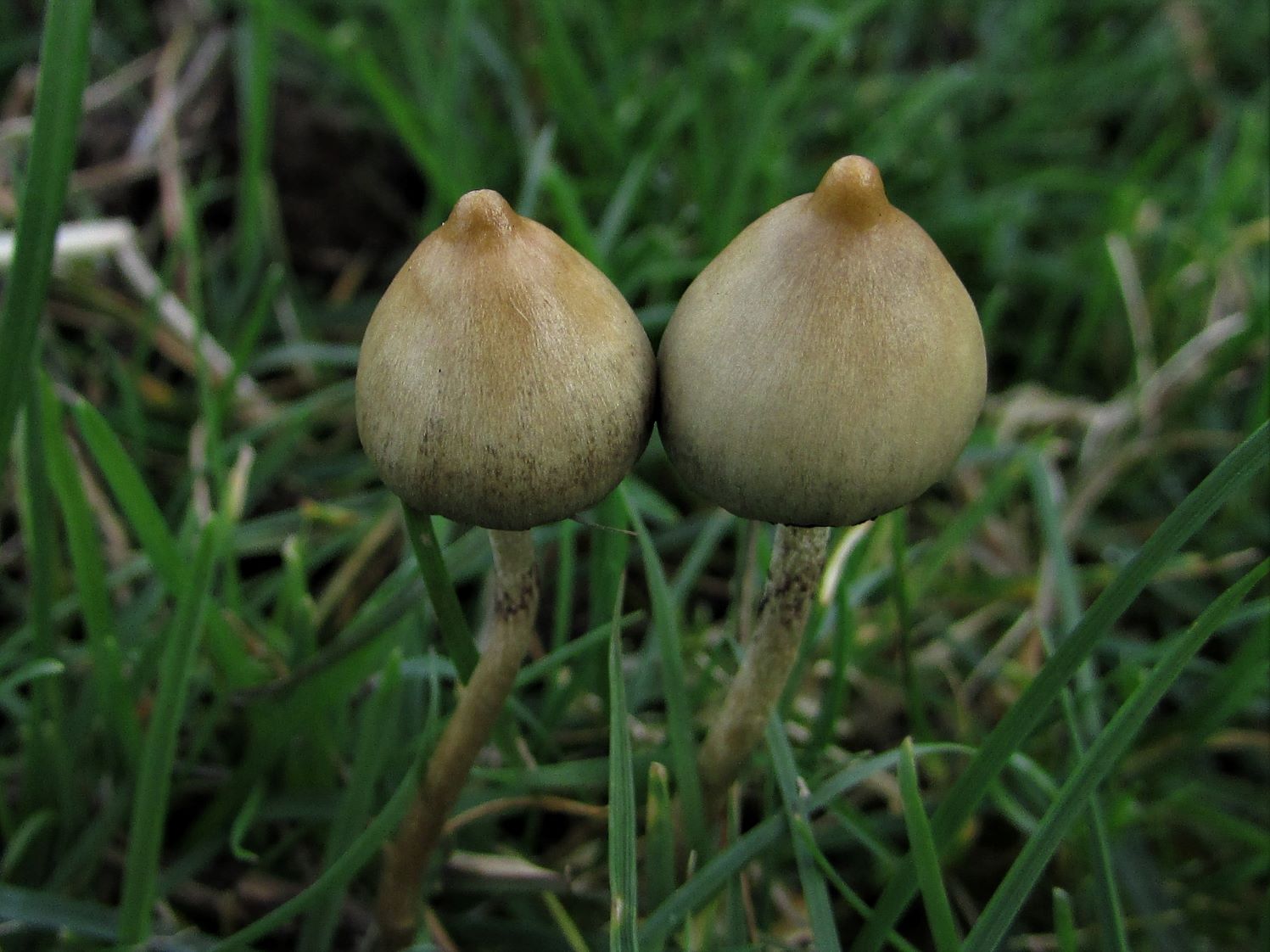This is a detailed, color photograph in landscape orientation, capturing two psilocybin mushrooms side by side in a grassy field. The mushrooms, emerging from a ground dense with grass blades that sometimes reach as tall as the mushrooms themselves, stand next to each other on curved stalks that lean slightly to the right before straightening upward. The one on the left is marginally smaller than its counterpart. Each mushroom has a round, bulbous cap with a slightly darker protrusion or bump in the center, lending a temple-like appearance to the top. The caps are fully enclosed, not yet developing into an umbrella shape, with a gradient in color from dark green at the stalk to light beige at the rounded peak. The image, in a style of photographic representationalism, captures the realistic and textured beauty of the mushrooms in their natural habitat.